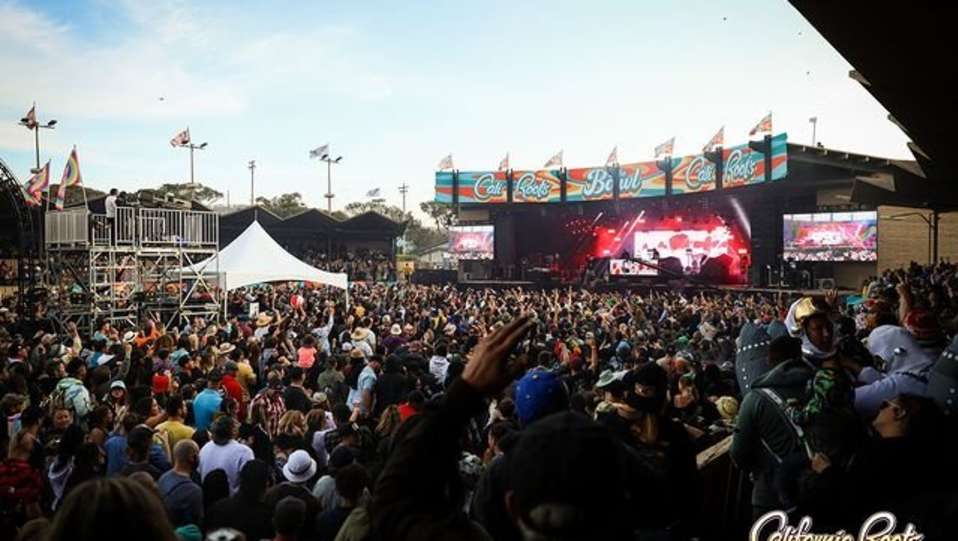This slightly blurry landscape photo depicts a vibrant outdoor concert under a sunny, slightly overexposed sky. The scene is dominated by a dense crowd, filling every inch of the standing-room-only venue, with attendees donned in a kaleidoscope of colorful outfits and hats. Their faces are indistinct as they face away from the camera, giving the impression of a sea of vibrant humanity. In the background, the stage is outfitted with bright red and white lights and flanked by large side screens, though the performers themselves are not visible from this distance. Above the stage, a curved marquee is partially readable, suggesting the name "Cali Rocks Bowl" or possibly "California Roots." To the left of the stage, a tall metal scaffolding platform stands high above the crowd, with flags fluttering in the wind and a figure, likely a cameraman, perched on top. Below the platform, a large white tent, reminiscent of a circus canopy, provides shade. Along the left edge, part of a building with a distinctive zigzag roof and stadium seating can be seen, adding to the festival atmosphere.